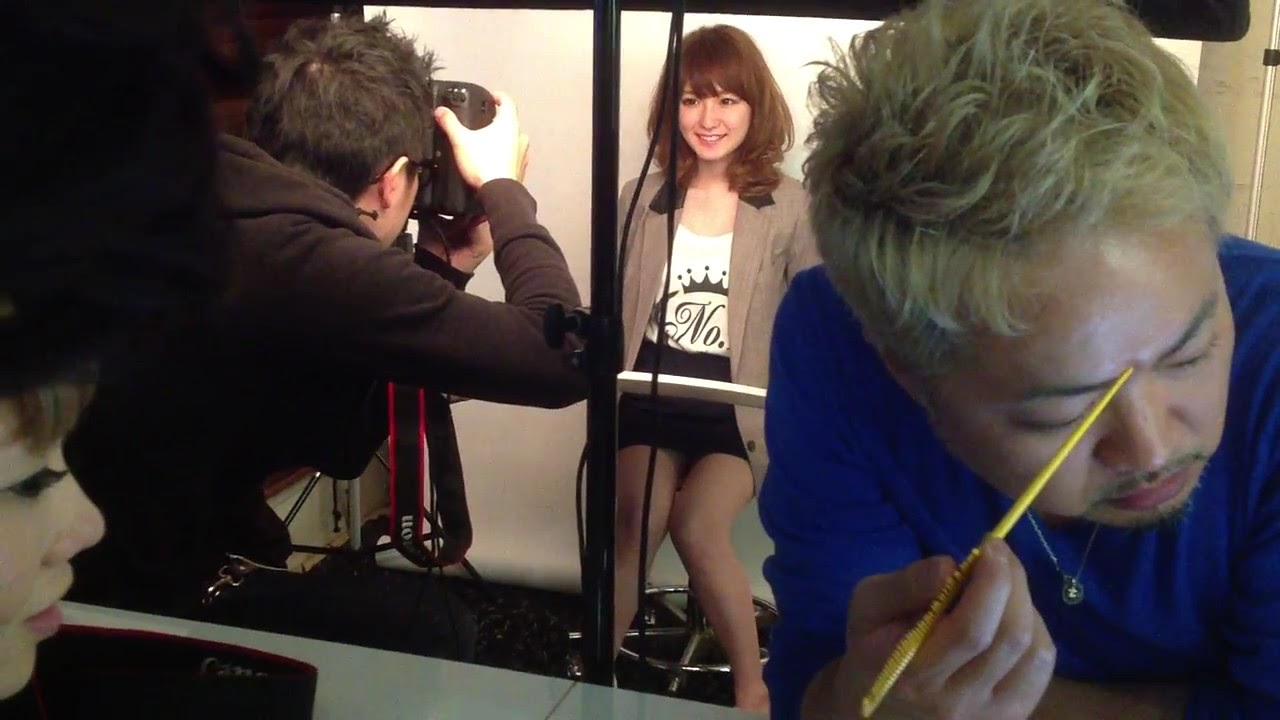In this lively photo shoot scene, an Asian woman is the focal point, seated on a stool at the center of the image. Her straight, shoulder-length brown hair with bangs frames her smiling face, and her light skin is illuminated by bright overhead lighting. She is dressed in a beige blazer over a white T-shirt adorned with a black crown and the letters "N-O." Below, she wears a black skirt, her legs together at the knees and slightly apart at the feet.

To the left side of the image, a man with dark spiky hair and a black hoodie captures her radiant smile with a camera, his back turned to the viewer. On the right side, the close-up profile of another Asian man with bleached blonde hair, parted to the right, focuses to his task. His face, adorned with brown eyebrows, closed eyes, a mustache, and a beard, is pointed downwards as he holds a golden paintbrush-like object between his eyebrows. This man wears a light blue shirt, adding a subtle touch of color to the scene.

In the bottom left corner, barely visible, is a hint of a female face with black artificial eyelashes, pink lips, and brunette hair peeking through. The backdrop of this busy photoshoot is a white sheet, adding to the professional ambiance, with artificial light casting a glow from above, likely from a pole that supports the lighting apparatus, partially cropped out of the frame. The scene is infused with a sense of dynamic artistry, capturing an intricate moment in the midst of a creative process.